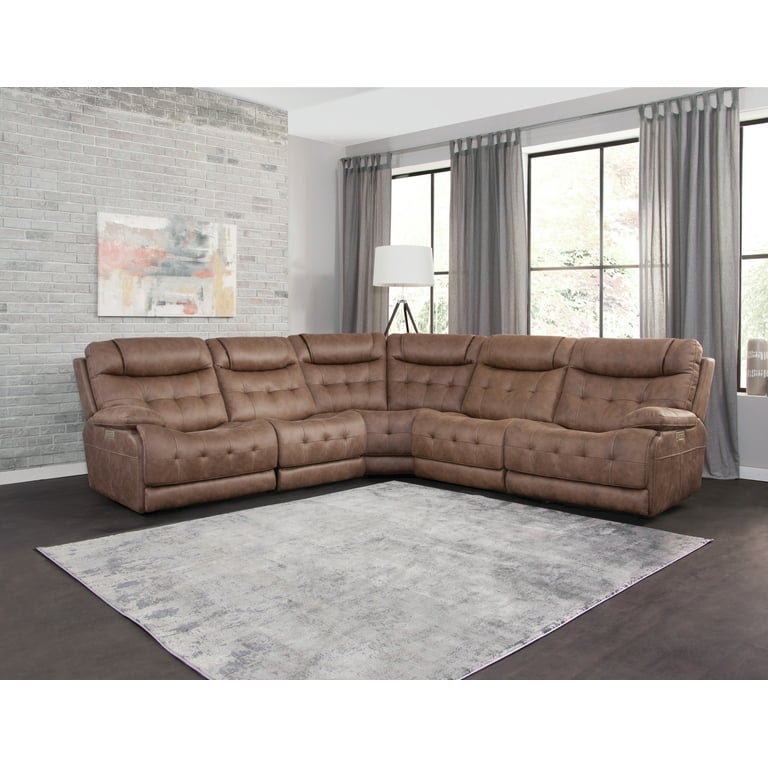This photograph showcases a stylish living room, possibly a model room or a product listing for furniture. The room features a large, brown leather sectional sofa positioned snugly in the corner, capable of seating about six people. Behind the sofa is a lamp with a white lampshade, providing soft lighting. The floor is a dark, hardwood surface with a light gray throw rug adding texture and contrast.

Dominating the walls are expansive windows framed in black, letting in ample natural light. Grey curtains hang elegantly from rods across the windows. One wall stands out with its white brick finish, peppered with gray bricks, adding a touch of rustic charm. Adorning this wall is an abstract watercolor painting with hues of pink, gray, and white, lending an artistic flair to the space. This modern yet cozy living room balances a mix of textures and neutral tones for a sophisticated look.